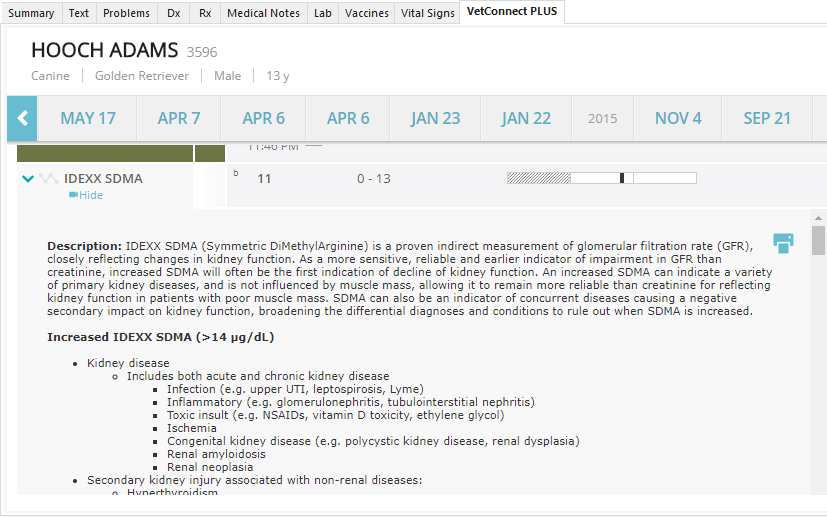**Detailed Caption:**

The image displays a digital medical record interface with a specific tab highlighted in white. At the top part of the interface is a horizontal tab navigation bar on a grey background. The tabs, labeled in black text, read from left to right: "Summary," "Text," "Problem," "Dx," "Rx," "Medical Notes," "Lab," "Vaccines," "Vital Signs," "Vets," and "Connect Plus," with "Connect Plus" being the highlighted tab in white.

Below the tab bar on the left side, there is a section that details patient information. The text states "Hook Adams 3596," identifying a "canine, golden retriever, male, 19." Underneath this identification, there are several dates listed in blue, ordered from most recent to oldest: "May 19," "April 7," "April 6," "April 6," "January 23," "January 2022," "2015," "November 4," and "September 21."

Further below, still on the left side, there is a heading labeled "IDEXX-SDMA" with a button beside it that reads "Height" in blue text, while the remaining text is in black. A detailed description follows, written in black, explaining the significance of IDEXX-SDMA (symmetric dimethylarginine) in assessing kidney function. The description denotes that SDMA is a proven indirect measurement of glomerular filtration rate (GFR), making it a more sensitive and reliable indicator of kidney function decline compared to creatinine. It is noted that increased SDMA can often be the first signal of kidney function impairment and is not influenced by muscle mass, making it a more consistent measure than creatinine. The description also highlights that elevated SDMA levels can indicate various forms of primary kidney disease and secondary conditions affecting kidney function, broadening the scope of differential diagnoses when SDMA is elevated. Conditions such as kidney disease, both acute and chronic, infections, inflammatory states, toxic insults, ischemia, cognitive kidney disease, renal amyloidosis, renal neoplasia, and secondary kidney injuries associated with non-renal diseases, as well as hyperthyroidism, are listed as potential causes of increased SDMA.